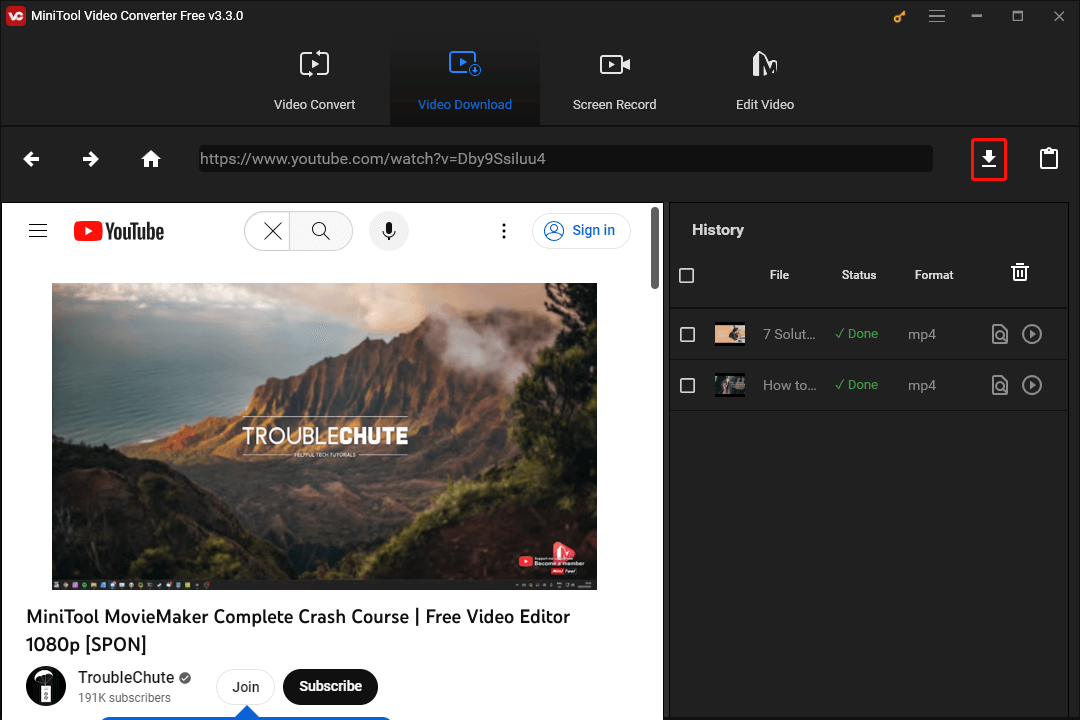This image is a screenshot from the MiniTool Video Converter software's interface, displaying its dark mode setting. The background is a very dark gray. In the upper left corner, the screen displays "MiniTool Video Converter Free" in white text, followed by the version number "V 3.3.0". Beneath this, a horizontal content menu lists several options: "Video Convert," "Video Download" (highlighted in blue font), "Screen Record," and "Edit Video" (all in white text).

On the lower left-hand corner, there's a large white background containing a web address for a YouTube video. At the top of this white square, the YouTube logo and text are visible, with the logo being a red square with rounded corners and a white triangle in the middle, symbolizing the play button. The thumbnail for the video features a stunning scene of a mountain with beautiful skies at either sunrise or sunset. The headline of the video reads "Troubleshoot," creatively spelled as "TroubleCHUTE." Below the headline, the title of the video is displayed: "MiniTool MovieMaker Complete Crash Course - Free Video Editor."